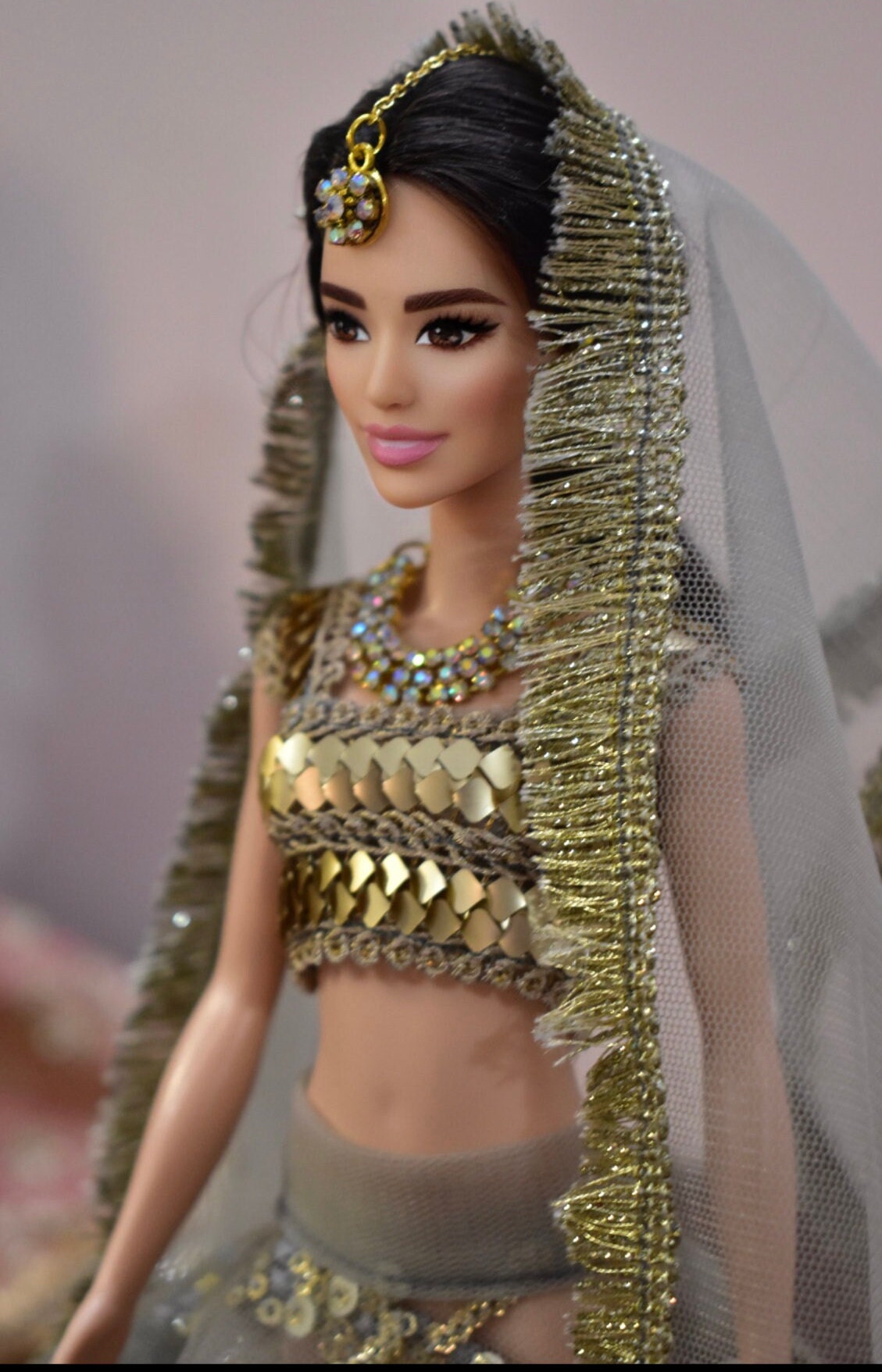The image showcases a Barbie doll with features reminiscent of Asian or Indian ethnicity. The doll is adorned in a gold belly dancer costume, featuring a gold bra top embellished with sequins and a gauzy material around the waist. She has dark hair styled under a gold and white veil that drapes over her head and shoulders, detailed with gold tassels along the edges. A prominent gold chain with a gemmed pendant hangs over her forehead, adding to her intricate jewelry. Around her neck are multiple necklaces, complementing her overall opulent look. The doll has dark eyes, pink lips, and dark eyebrows, enhancing her striking appearance. The background is a blurry light gray-pink color, placing emphasis on the beautifully dressed doll in the foreground.